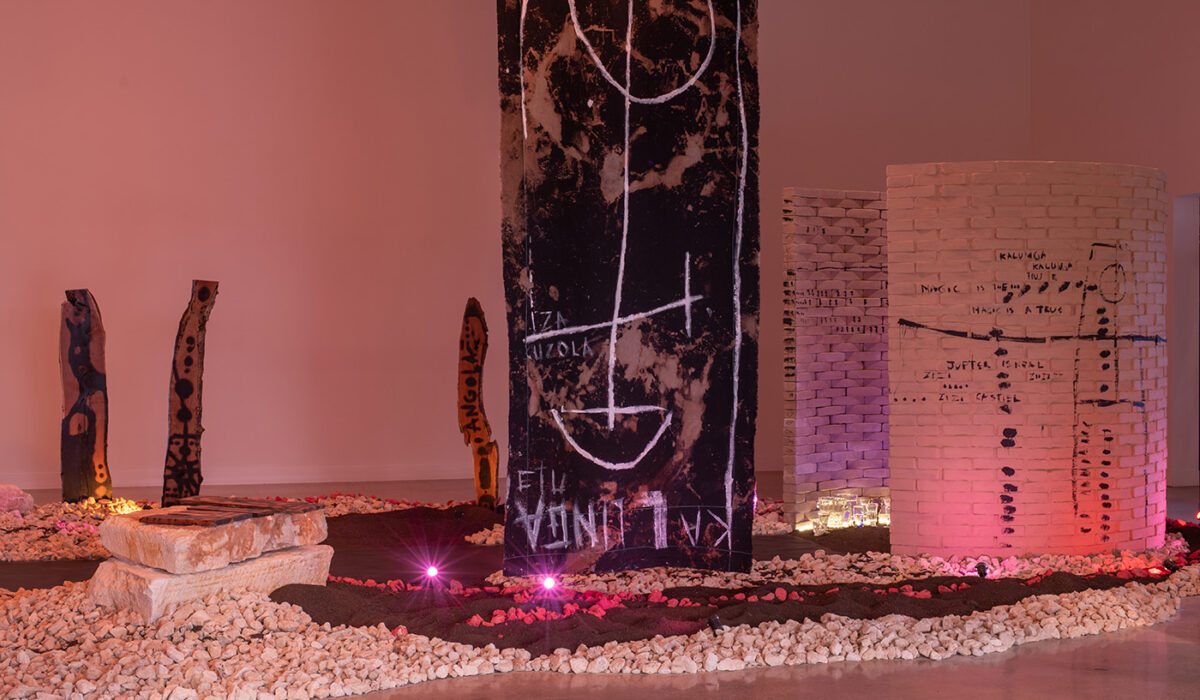The image showcases an indoor art exhibit, specifically the Andrew Warhol art exhibit titled "Social Fabric for Art and Activism." The setting features a white wall and a linoleum floor adorned with white-beige gravel. In the center, there is a large weathered black stone with gray and beige streaks, covered in white chalk graffiti. The graffiti includes a complex drawing of a circle with intersecting lines, and upside-down text that possibly spells "Kalunga." 

Surrounding the central stone are multiple sculptures and structures set atop the gravel. These include various smaller stones and tablets with black writing and diagrams, reminiscent of ancient artifacts or text-laden art pieces. Each sculpture is highlighted by pink lighting, adding a vivid contrast to the otherwise monochromatic setting.

To the right, there is a circular brick wall with an opening that emits a white light. The exterior of this wall features additional black graffiti, including black dots, lines, and possibly crude depictions of buildings. On the left, two stone tablets, resembling the Ten Commandments in shape, stand upright with black inscriptions. Overall, the exhibit merges elements of art, activism, and obscure symbolism under an ethereal pink illumination.